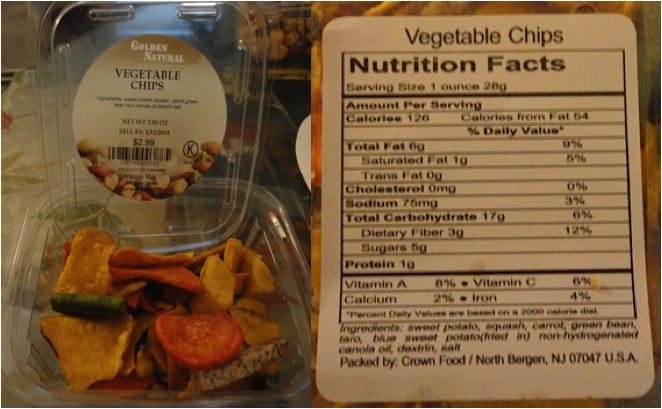The image showcases a vibrant assortment of vegetable chips in a partially opened container. The variety of chips, in shades of green, red, yellow, and subtle gray at the bottom, create a colorful display. The container's lid, which is also open and resting inside the contents, bears a vivid label.

The circular label prominently reads "Golden Natural Vegetable Chips" in a white font against a brown background at the top, with the other details in black text on a white backdrop. The net weight of the package, 3.5 ounces, along with the barcode, the sell-by date of 1-11-2014, and the price of $2.99, are visible. A notable feature on the left side of the label is the letter "K". Below, encircling about a third of the bottom portion of the label, are images of the vegetable chips themselves.

On the left side of the image, a rectangular box displays the nutrition facts. In clear, black text, it states:

- Serving Size: 1 ounce
- Calories: 126 (with 54 calories from fat)
- Total Fat: 6 grams (9% of daily value, DV)
- Saturated Fat: 1 gram (5% DV)
- Trans Fat: 0 grams
- Cholesterol: 0 milligrams (0% DV)
- Sodium: 75 milligrams (3% DV)
- Total Carbohydrates: 17 grams (6% DV)
- Dietary Fiber: 3 grams (12% DV)
- Sugars: 5 grams
- Protein: 1 gram

Additionally, the vitamins and minerals content includes 8% of daily vitamin A, 6% of vitamin C, 4% of iron, and 2% of calcium. This nutritious snack is crafted by Crown Food, based in North Bergen, New Jersey.